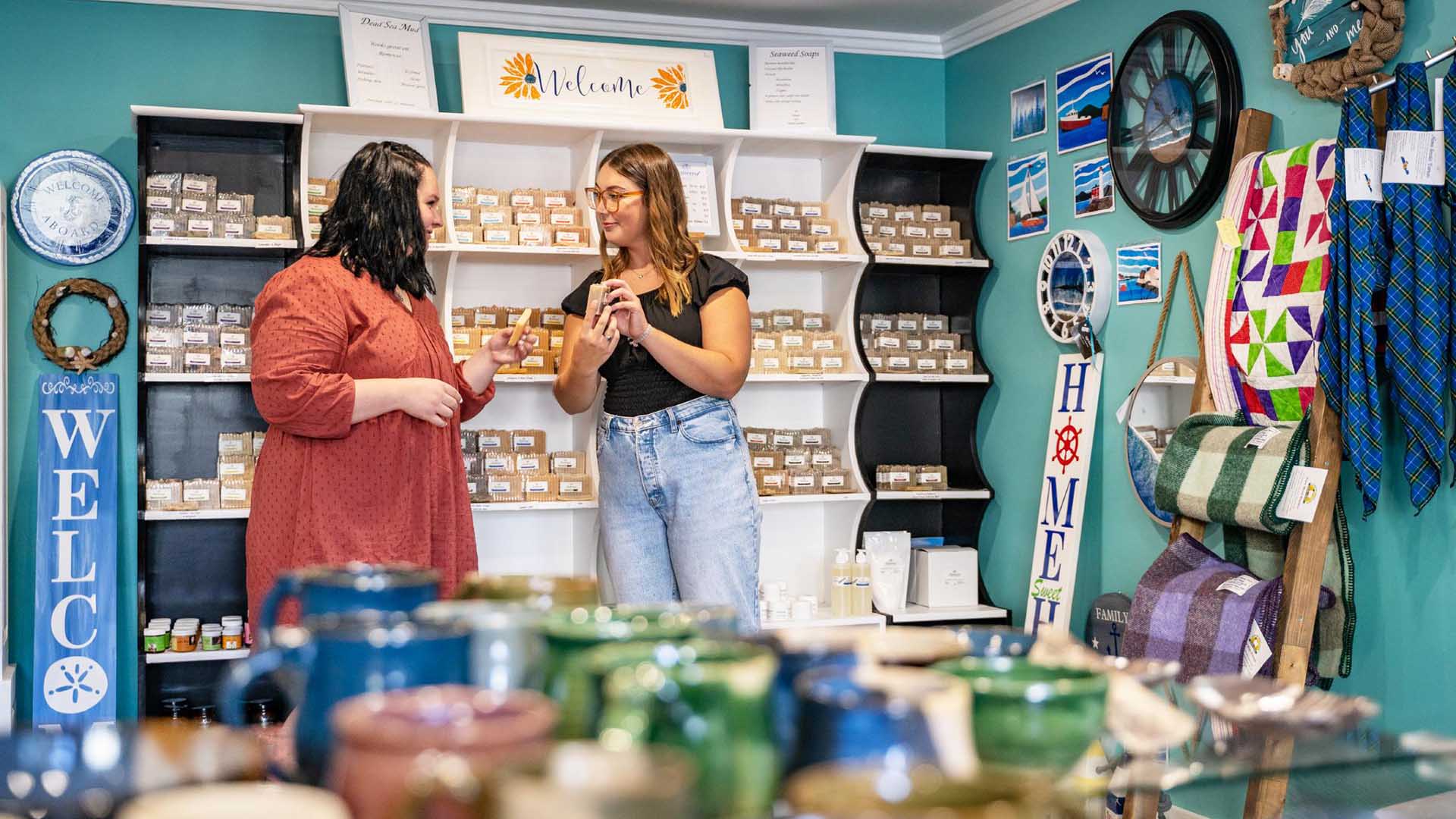In the image, two women stand behind a glass table, set before a cubby-style rack full of various shades of brown and yellow slabs or boxes, each adorned with a white label. The women appear to be selling handmade soap. The table in front is cluttered with an array of small ceramic objects, predominantly mugs, with one small bowl. On the right wall, three quilts hang on a rack alongside what appear to be plaid scarves. 

A distinct blue hanging on the left reads "WELCOME," though the text is slightly clipped and features a sand dollar representing the "O." The booth, set against turquoise walls with white trim, showcases the women who are selling handcrafted items. One woman, slightly heavy-set, wears a red calico dress and has dark, almost black hair. The other woman, with lighter brown hair possibly highlighted, wears glasses with brown rims, a black top with extremely short or "butt" sleeves, and faded blue jeans. 

Both women are engaged in conversation, holding small products—a white and orange package and a brown box. Surrounding the scene are further nautical and home-themed decorations, including signs that say "Home" with a captain's wheel for an "O" and assorted decorative pieces. The store exudes a gift shop ambiance, brimming with handmade and nautical-themed items.